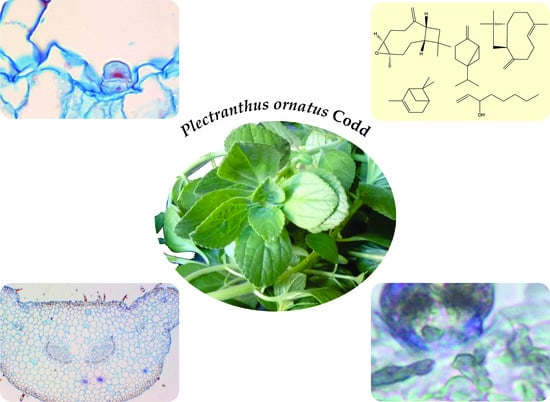The image features a central picture of a green plant, labeled "Plectranthus ornatus cod" in black text above it. Surrounding this middle image are four corner images, each showcasing different scientific visuals. The top left corner displays a pink-tinted microscopic view with intricate blue lines, reminiscent of microorganisms on the leaf. The top right corner contains various geometric shapes like polygons and hexagons, suggesting chemical structures or molecular diagrams. The bottom left corner presents a detailed close-up of cellular or atomic structures, appearing as interconnected circles. The bottom right corner offers another zoomed-in biological view, filled with vibrant blues, pinks, and greens. The background predominantly remains white, drawing focus to the intricate and colorful scientific imagery around the central plant.